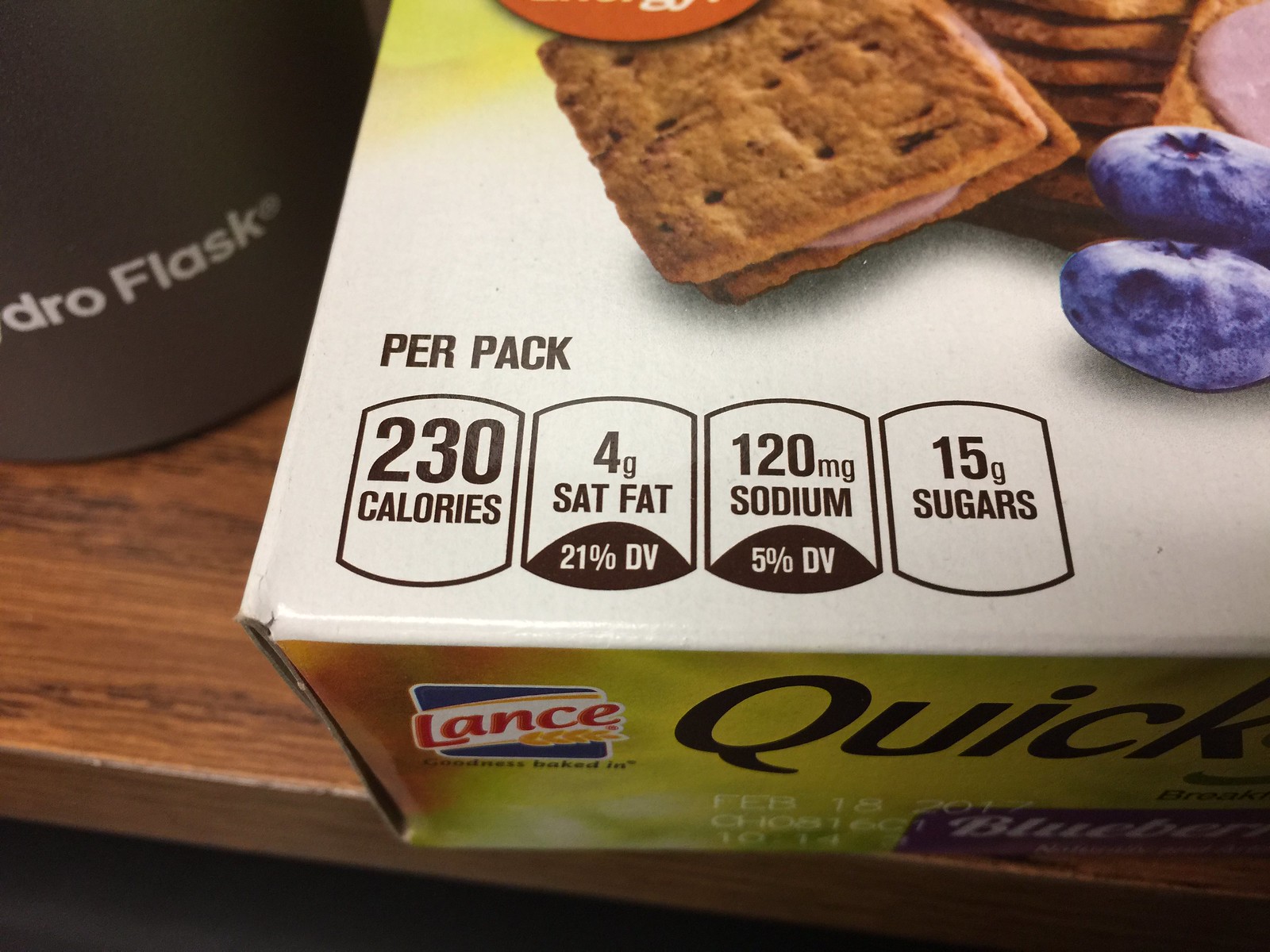This detailed image captures the corner of a box of Lance brand crackers placed prominently on a wooden tabletop with a light horizontal grain. The box occupies about three-quarters of the photograph, with its sides aligned to the upper and right edges. In the upper left corner of the image, a gray Hydro Flask bottle, with its white logo clearly displayed, adds to the scene. The box itself features a white cover adorned with images of square tan biscuits sandwiching a pink cream filling, stacked neatly. Complementing the crackers are two blueberries positioned in front. The side of the box is yellow, displaying the Lance logo, the word "Quick," and a blue bar with white text reading "Blueberry." Nutritional information is visible on the lower left corner of the box, listing 230 calories per pack, 4 grams of saturated fat (21% daily value), 120 milligrams of sodium (5% daily value), and 15 grams of sugar.